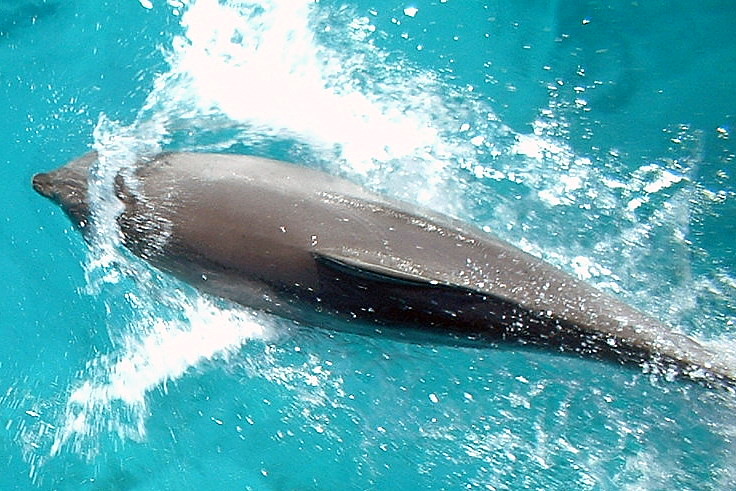This vibrant, full-color photograph captures a dynamic scene set in the outdoors, possibly in the ocean or at a theme park, during daylight. The main focus is a lively dolphin gracefully leaping through the air, creating a splash that disturbs the otherwise deep, rich blue water with splashes of white. The dolphin, gray in color with darker shading on its lower body, shows off its distinctive dorsal fin and nose prominently. The image highlights the dolphin's movement from left to right across the center, emphasizing the lively, turquoise-blue water and the energetic white splashes. Despite the clear visibility of the dolphin’s upper body, its back flippers and tail are not visible.